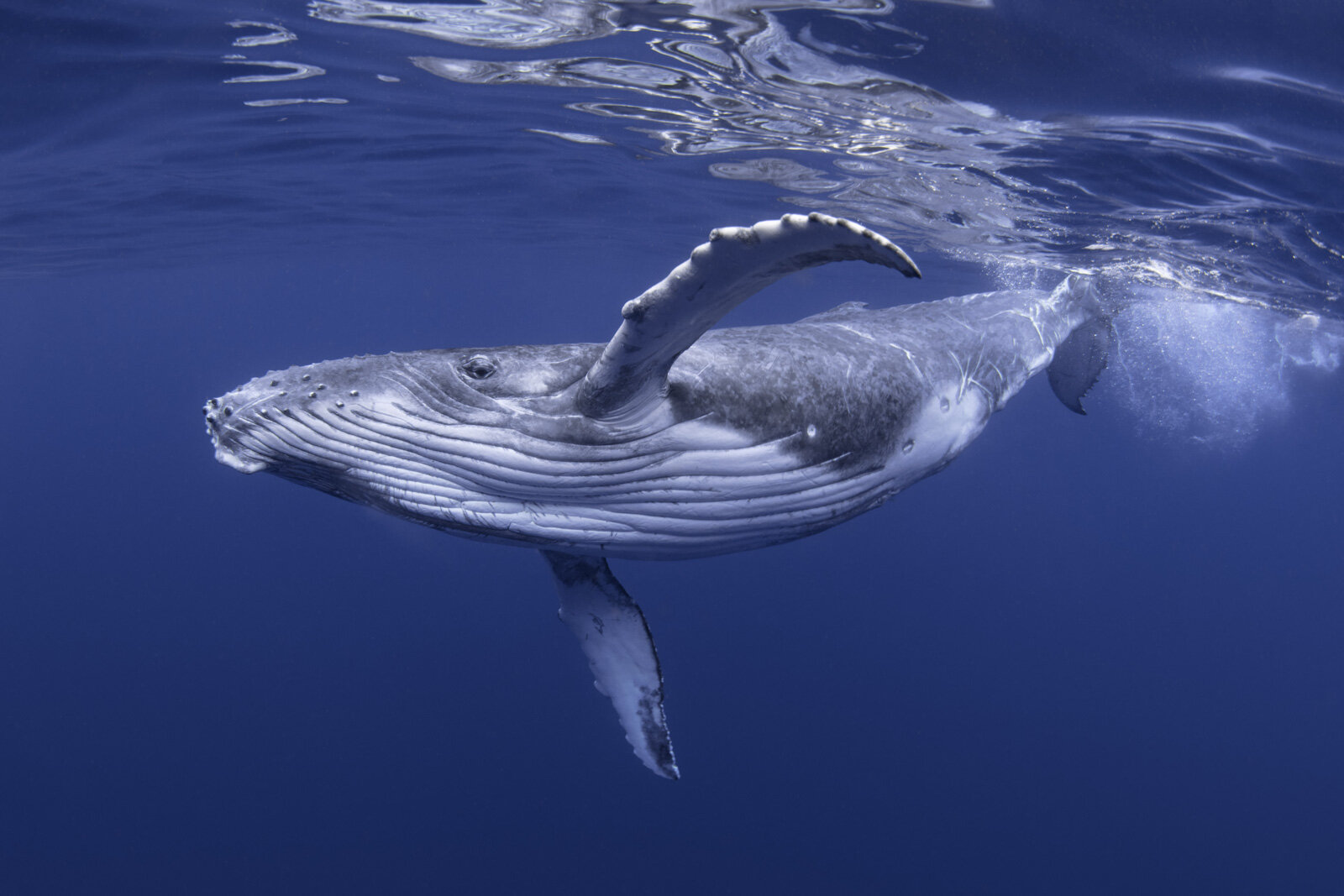This horizontal, rectangular image depicts a majestic blue whale in motion underwater, caught mid-swim with its substantial, textured fins appearing to flap and move. The whale's large body is primarily a dark gray, accented with light gray patterns and small textured spots, especially on its underside. Its eye, positioned toward the back of its long face, is open, while its mouth remains closed. The scene is bathed in a perfect ocean blue, almost navy, with light ripples and bubbles visible throughout the water, possibly indicating the whale's recent movement. The sunlight creates shimmering effects and faint shadows on the water surface, adding to the image's striking clarity and almost surreal quality, suggesting it might be a computerized depiction. Notably, there are no other fish or any additional marine life present in the scene, and no details hint at a specific date, time, or location.